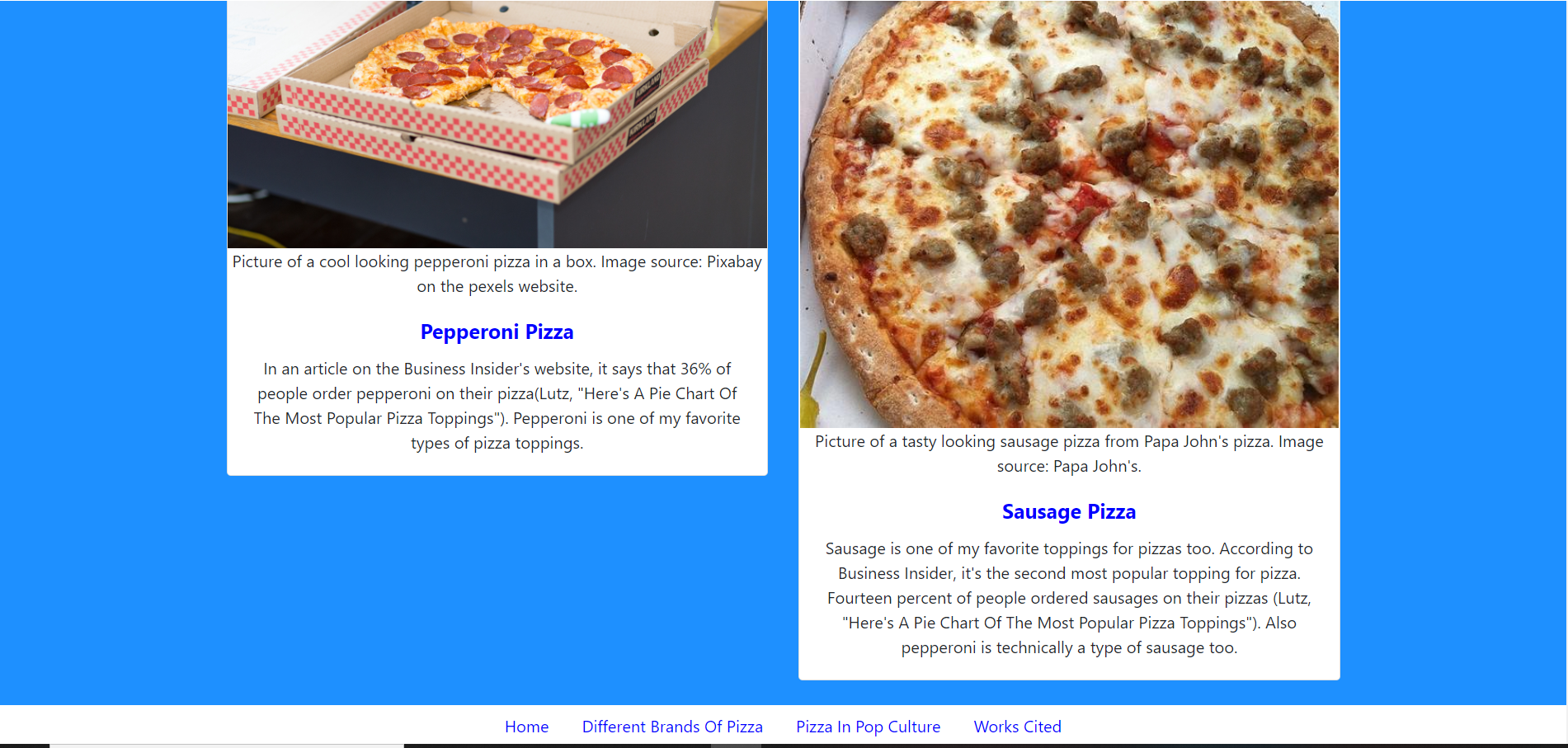The image features a light blue background and contains two distinct boxes, each with a photo at the top and text below. 

**Left Box:**
- **Image Description:** The photo displays three boxes of pizza. One pizza box is open and stacked atop the other two, showing a pepperoni pizza with one or two slices missing.
- **Image Source:** Pixabay on the Pexels website.
- **Headline in Blue:** "Pepperoni Pizza"
- **Text Below (in Black):** "In an article on the Business Insider website, it stated that 36% of people order pepperoni on their pizza. (See pie chart of the most popular pizza toppings.) Pepperoni is one of my favorite types of pizza topping."

**Right Box:**
- **Image Description:** The photo shows a sausage pizza with cheese, looking appetizing.
- **Image Source:** Papa John's website.
- **Headline in Blue:** "Sausage Pizza"
- **Text Below (in Black):** "Sausage is one of my favorite toppings for pizza, too."

The overall presentation is visually neat, separating the two captions effectively and providing a clear, engaging overview of the pizza types and personal preferences.